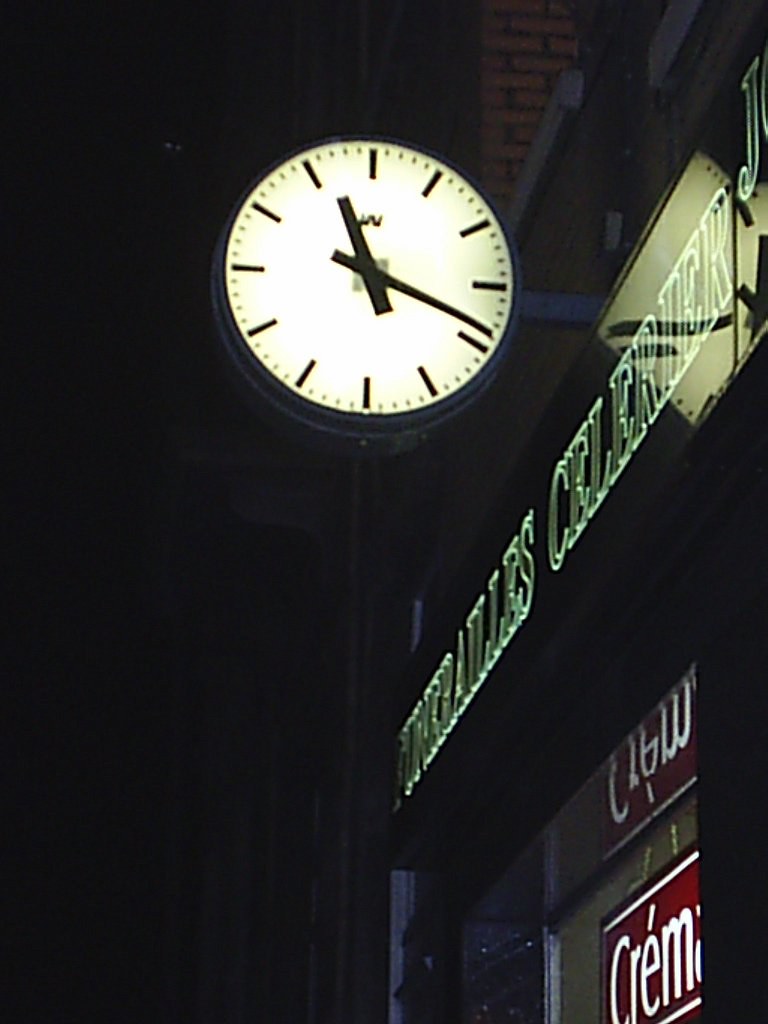This color photograph taken at nighttime depicts an illuminated storefront set against a dark, starless sky. The focus is on a circular clock, which hangs from an arm extending out from the building. The clock, surrounded by a blue frame, is illuminated with a white face featuring black hands and dashes in place of numbers, indicating that the time is 11:19. Below the clock, green neon lights illuminate the shop's signage, which is partially obscured and unreadable. Further below, through the storefront window, there's another sign in red with white writing that reads "CREMA," though the rest of the sign is cut off. The overall scene exudes a quiet, nighttime ambiance with the neon and clock being the primary sources of light.